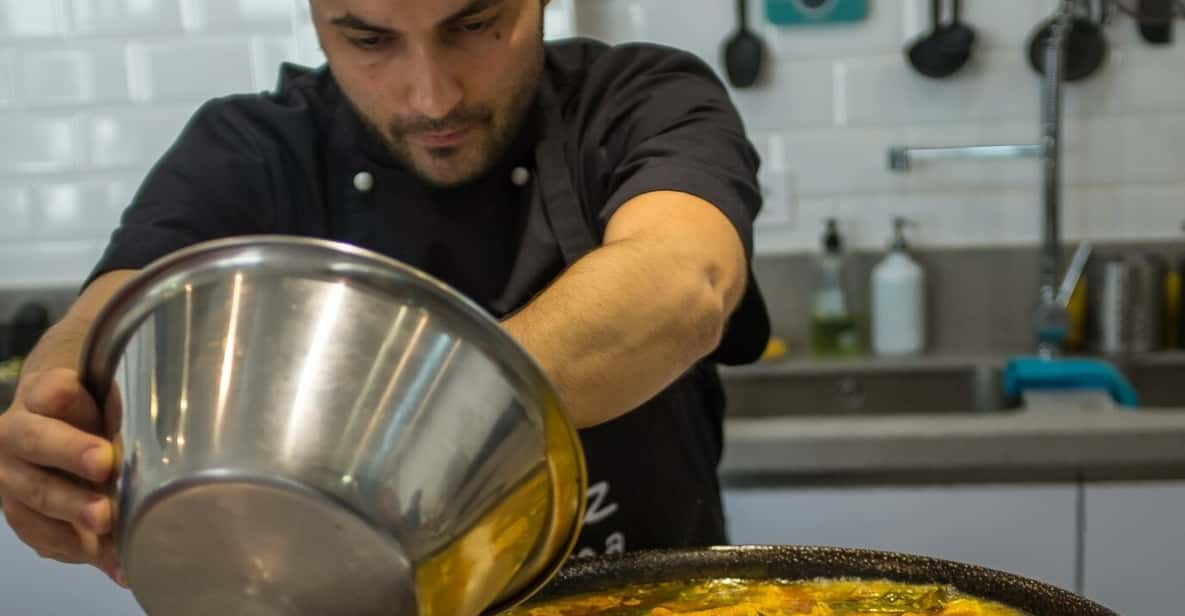In the kitchen, a man with dark hair, a mustache, goatee, and beard stands focused and serious. He is dressed in a black button-up shirt and a black apron featuring two white buttons at the top, obscuring any text or smaller details. The man is holding a rounded, metallic bowl in his right hand, while his left hand is engaged inside the bowl, indicating he is preparing a dish. A frying pan with oil is positioned next to him, ready to be used. Behind him, the kitchen features a white Subway-tiled backsplash and a sink area with a green soap bottle with a black top, a white soap bottle with a silver top, and an upside-down cup. Above the sink, black spoons hang on the wall. A blue dish rag is laid out on the gray countertop, contributing to the well-used and practical atmosphere of the kitchen.